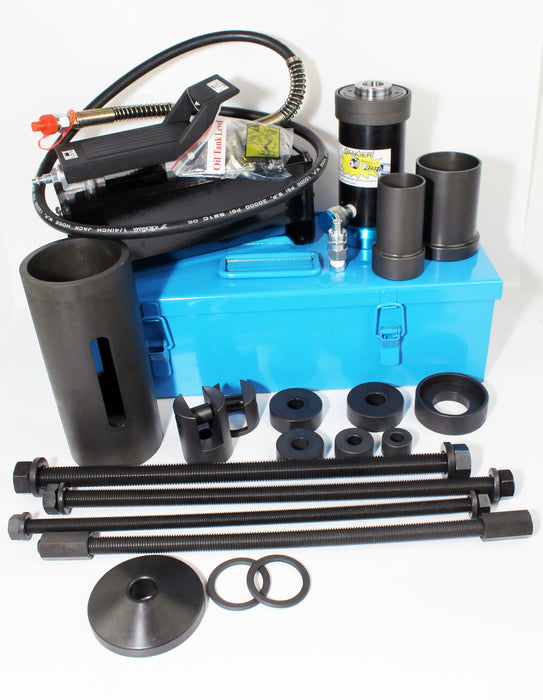The picture displays a light blue rectangular metal toolbox with metal clasps. On the top left of the box, there is a black wire with silver ends, coiled neatly. Adjacent to this, on the right-top of the box, are three black and grey cylindrical objects, one of which features a red cap and resembles a pump. The box's latches are flipped up, revealing detailed components. In front of the toolbox, on the left, stands a taller black cylindrical tube with a large oval indentation, indicating it might be hollow. On the right, there are smaller black wings, and in front of these wings are four black poles with screws at the ends, next to silver washers. A pair of interlocking rings rests alongside these items, all set against a light gray background.